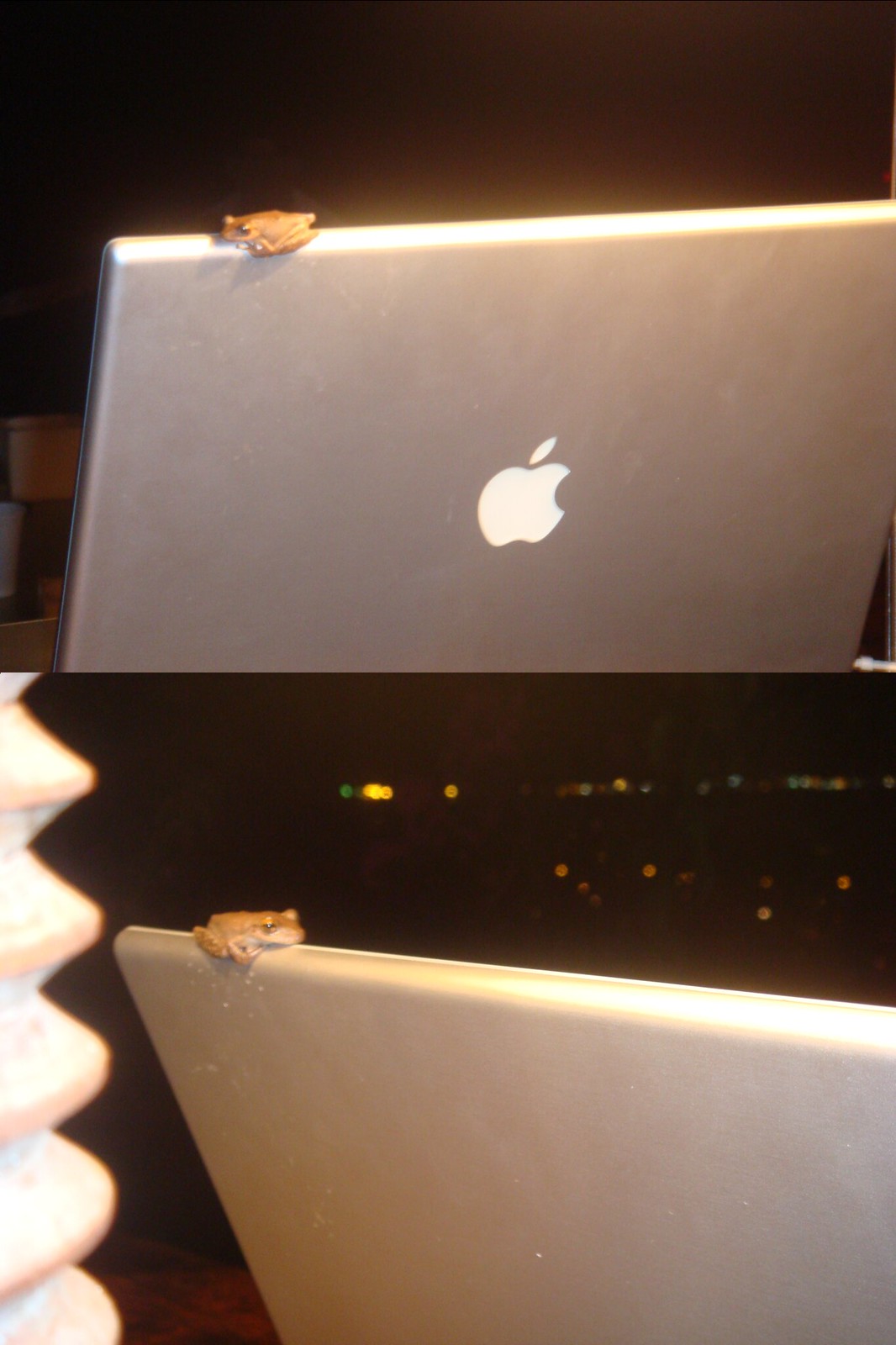This intriguing nighttime image appears to be taken outdoors and shows a unique, dual-perspective composition that almost resembles a collage. At the top of the picture, a sleek, silver Apple MacBook is prominently displayed, with its iconic glowing Apple logo in white visible from the back. Perched on the edge of the MacBook is a tiny, orange-brown baby frog. The bottom portion of the picture presents a different angle of the same scene, featuring the MacBook and frog from another perspective. Here, the frog is seen hanging out on the opposite side of the laptop's lid. The background is dark, suggestive of an evening or nighttime setting, and distant city lights and the outline of a building’s wooden table or wall can be discerned towards the left side of the frame. The juxtaposition of the frog with the high-tech MacBook amidst an urban nightscape creates a captivating and whimsical visual narrative.